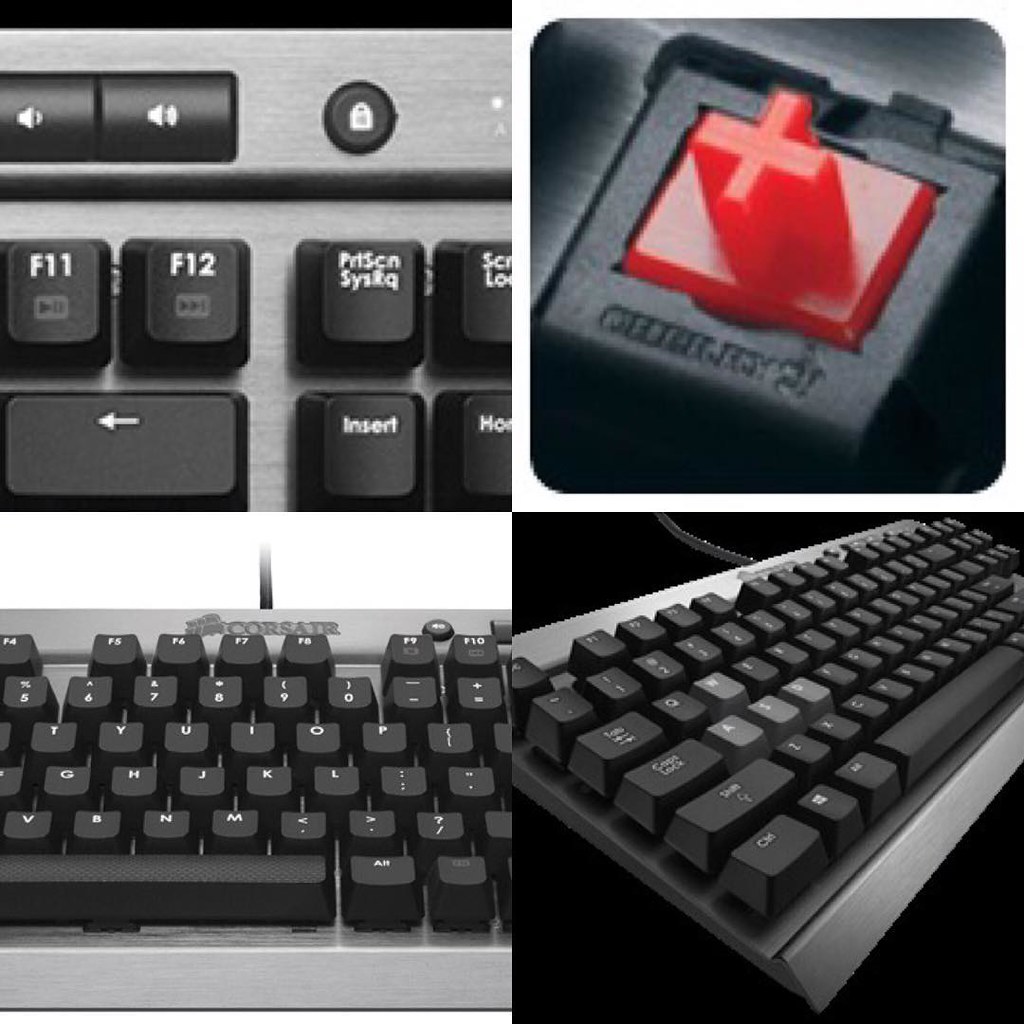This composite image consists of four photographs arranged in a grid, showcasing various views of the same gray and black Corsair keyboard. The top-left image provides a close, top-down view featuring the F11, F12, Print Screen, and volume control buttons. The adjacent top-right image displays a close-up of a unique button with a raised red 3D plus sign, which may function akin to a joystick or a special input device. The bottom-left photograph highlights the Corsair logo and presents a front view encompassing keys from the middle of the space bar to the F10 key. The final bottom-right image gives an angled left-to-right perspective of the keyboard with jagged edges, possibly edited in Photoshop, and reveals a cable extending from the back. The black background creates the illusion of the keyboard floating in mid-air, emphasizing the keyboard's vintage design with large, raised keys and white lettering.